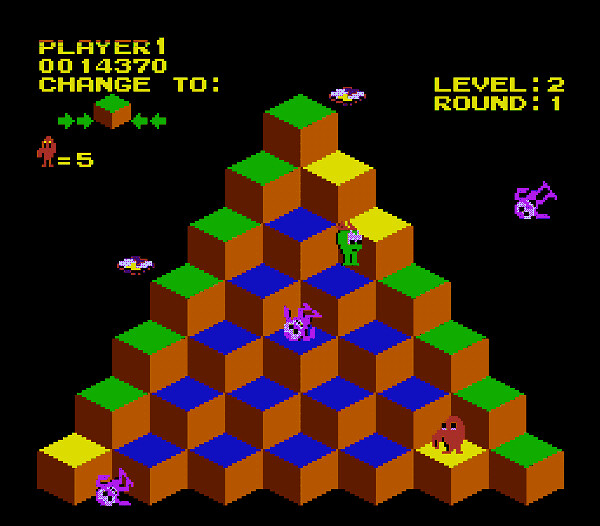The image depicts a classic arcade game from the Atari era, capturing the nostalgic charm of early gaming. The background is predominantly black with vibrant colors defining its elements. At the top of the screen, a red banner is featured, standing out against the mostly yellow interface. Just below, "Player One" is displayed in yellow text, accompanied by the score "0014370."

Beneath the score, instructions for game mechanics are indicated: "Change to..." followed by a series of four green arrows, two on each side. The central focus of the display is a large, pyramid-style arrangement of cubes. The cubes are intricately detailed with two brown sides and a differently colored top surface – variations include blue, green, and red.

Scattered around the pyramid are pixelated monsters of different colors, adding to the game's challenge and visual appeal. These monsters are depicted in shades of purple, green, and brown, some of them appearing to tumble down the sides of the pyramid. The overall layout and design elements strongly evoke the visual and gameplay aesthetics of early Atari games.